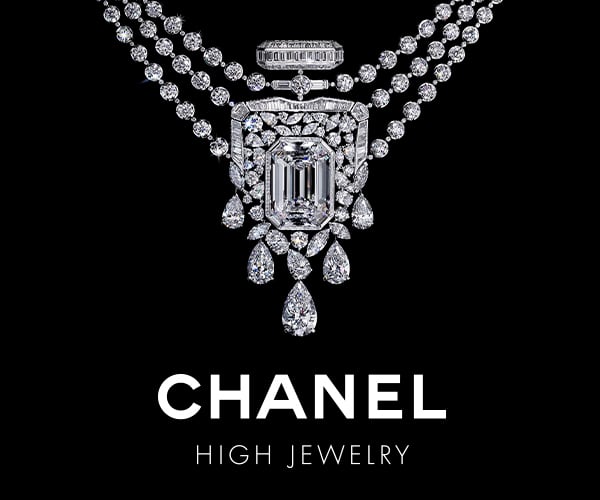The image is a striking advertisement for Chanel High Jewelry set against a solid black background. Dominating the center is a luxurious necklace featuring three diamond-studded chains. At the focal point is a grand, shield-shaped pendant adorned with a multitude of small diamonds and a prominent, large central diamond. Hanging from this intricate pendant are six smaller, teardrop-shaped diamond pendants, creating a cascade of shimmering brilliance. Completing the sophisticated layout, the bottom of the image displays the Chanel branding in large white all-caps text, with the phrase "High Jewelry" in a smaller, elegant white font beneath it. The overall composition exudes elegance and opulence, highlighting Chanel's exquisite craftsmanship in high jewelry.